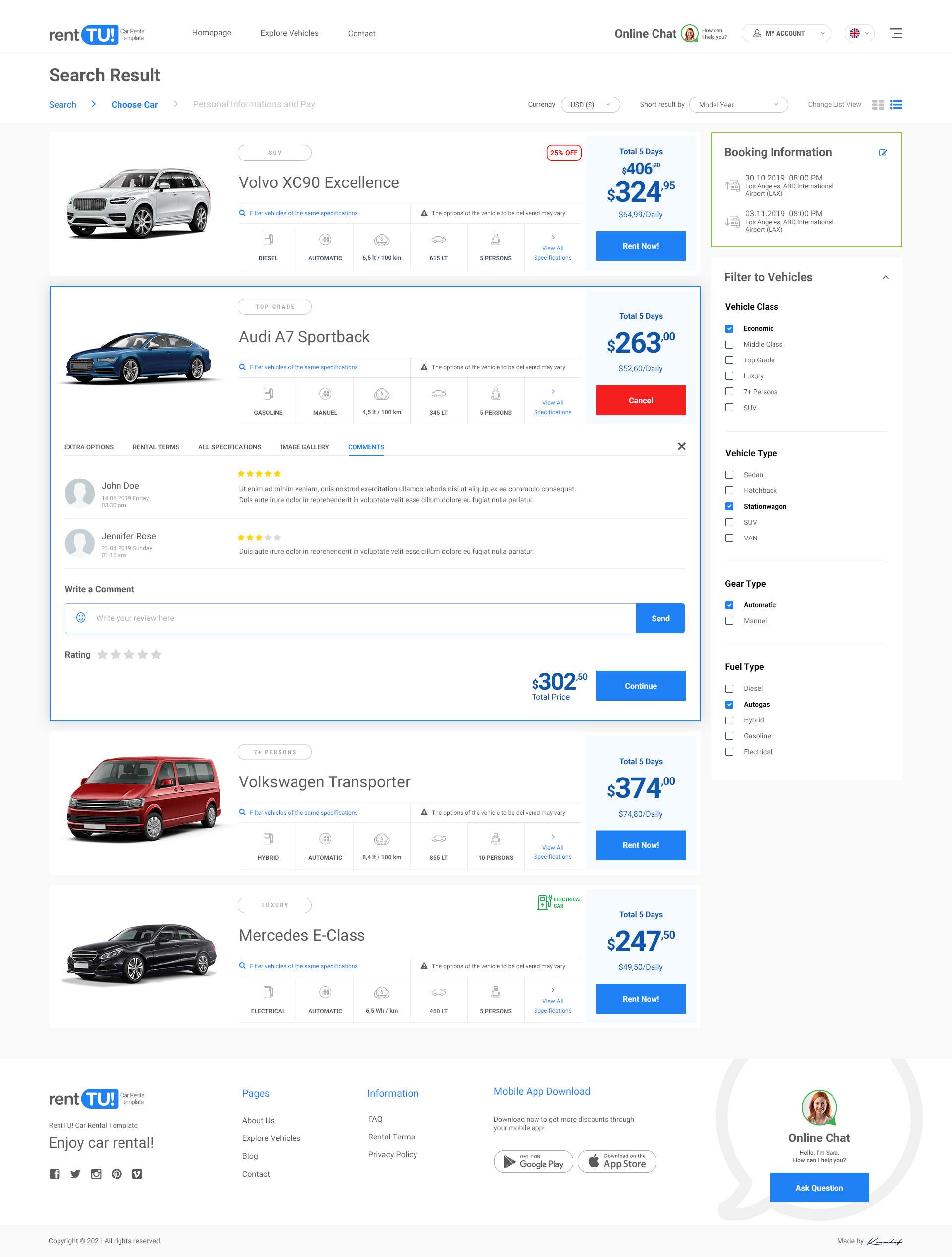**Caption:**

The image showcases a car rental website with a vibrant blue background. Titled "Rent 2 U", this platform offers an intuitive interface for renting cars. The top left corner prominently displays the brand "Rent 2 U". The homepage navigation includes links to "Homepage", "Explore Vehicle", "Contacts", and "Online Charts". The top right corner features links for "My Account", "Language", and "Options".

The main section of the page contains "Search Results", with categories for "Search", "Choose Car", "Personal Information", and "Pay". Users can sort results by various criteria, including currency and the monthly or yearly basis. There is a feature to change the list view as well.

The first menu item displays a Volvo X90 Excellence, a silver car with a 25% discount – indicated by red text. The rental price is noted as $24.95 for five days, with a daily rate of $64.99. Key specifications include its diesel automatic engine, fuel efficiency of 6.5 litres per 100 km, 650 pound-feet torque, and capacity for 5 passengers. A "Rent Now" button is prominently featured in blue, along with an option to view all specifications.

Highlighted centrally is the Audi A7 Sportback, in blue, featuring a manual transmission and gasoline engine with a consumption rate of 4.5 litres per 100 km, and a 45-litre boot space. It can accommodate 5 passengers and includes extra options like rental terms, an image gallery, and comments. User reviews are shown, written by John Doe and Jennifer Rose, with a space to write new comments and a "Send" button. There's a "Continue" button for confirming the rental, with the car priced at $2.

Below these listings are additional options: a Volkswagen Transporter priced at $3.74, and a Mercedes E-Class at $247.5. 

The footer of the website provides links to key sections such as Pages, Information, Mobile App Download, Tax, Rental Terms, Privacy, Blog, Contacts, and Pro Vehicles. The bottom left corner features the motivating message "Enjoy Your Rental Car".